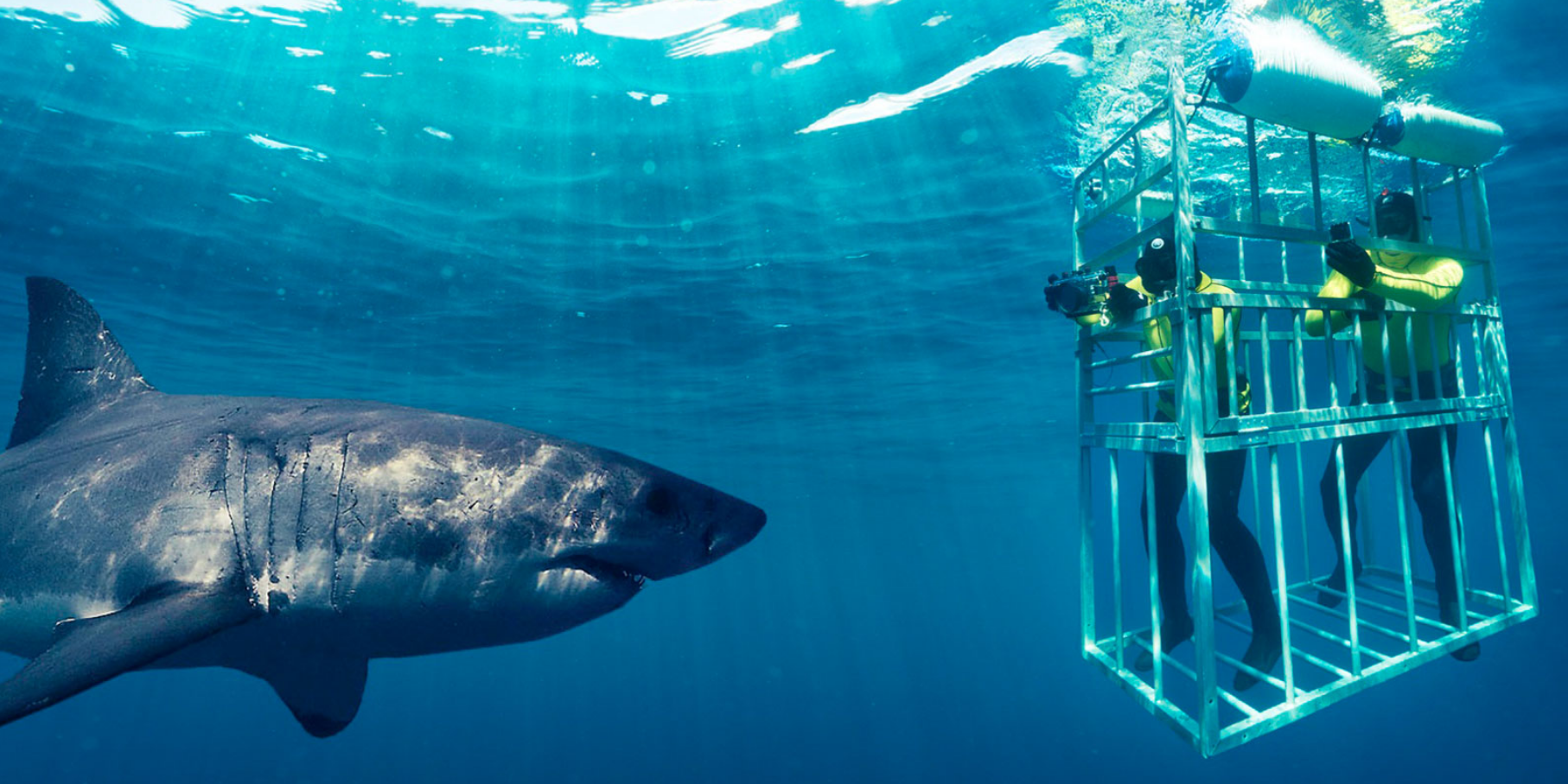This underwater photograph captures a mesmerizing scene with a gradient of deep blue at the bottom transitioning to a blue-green hue near the surface. Sunlight pierces through the water, creating striking rays that illuminate the entire setting. On the left side of the image, a sleek gray shark is visible, distinguished by its darker facial area, lighter belly, and darker fins. The shark's gills are prominently striped, adding to its majestic appearance. On the right side, a blue cage containing two scuba divers stands out. Each diver is equipped with a camera in an underwater case, dressed in black pants and bright, reflective green shirts. Their presence adds a human element to this vibrant and dynamic underwater tableau.